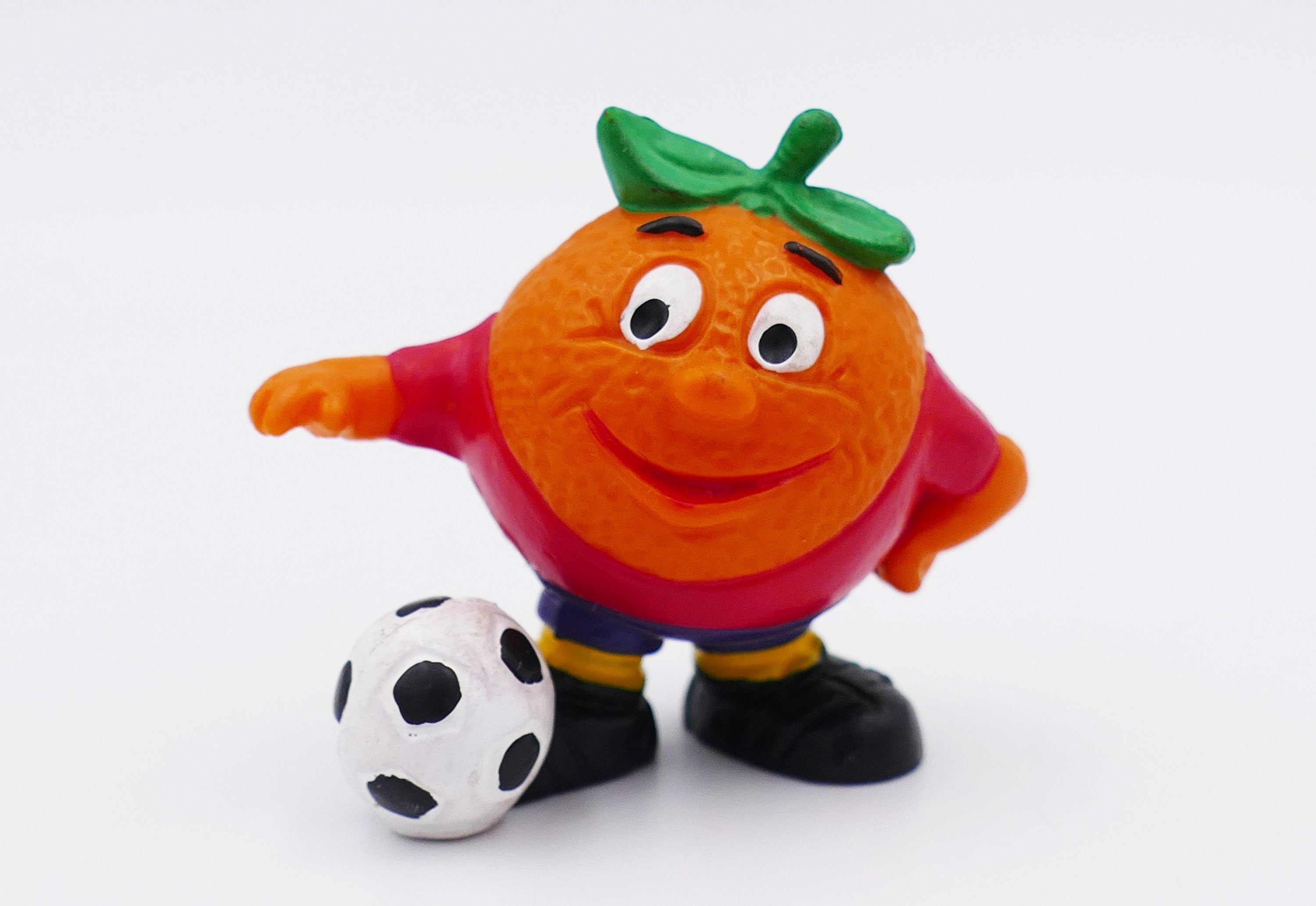The image features a children's toy designed to look like an animated character, specifically an anthropomorphic orange. This toy, which resembles a plastic figurine, is positioned centrally in the image, displaying a bright and lively color palette including orange, green, red, blue, yellow, black, white, and grayish white. The toy itself is stylized with big black and white eyes, black eyebrows, and a smile. It is dressed in a pink shirt, blue pants, yellow socks, and black shoes. Atop its head is a green leaf reminiscent of a hat, akin to a green beret. The orange's right hand is lifted and bent at the elbow, resting on its hip, while its left hand is extended outward. By its left foot lies a black and white soccer ball. The character is depicted standing on a white surface against a plain white background, giving it the appearance of being ready to engage in playful activity. This setup evokes the style of a children's cartoon or a toy from a children's television program or movie.